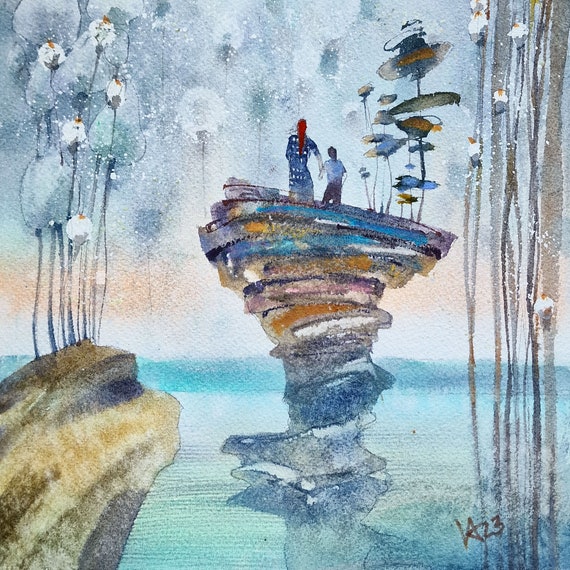The image appears to be a scan or photograph of a surreal painting. At the bottom, there is a lake or a similar body of light blue or turquoise water. Central to the composition is a towering, twister-like rock formation painted in a blend of blues, purples, oranges, and tans, with touches of white. Atop this rock stand two figures: a woman on the left, who has long red or purplish hair and wears a blue and white dress, holding hands with a boy on her right, who is in a blue shirt and dark pants. This rock outcrop also features peculiar trees or mushroom-like growths with thin stems and flat, colorful tops in shades of blue, orange, and brown. Surrounding the scene to the left and right are long-stemmed flowers emerging from the water, characterized by dark stalks and white petals with yellow dots in the center. In the bottom left corner, there is a more traditionally-colored tree with brown and gray hues. Additionally, the bottom right corner of the image contains "ka-23," likely the artist's signature or initials.